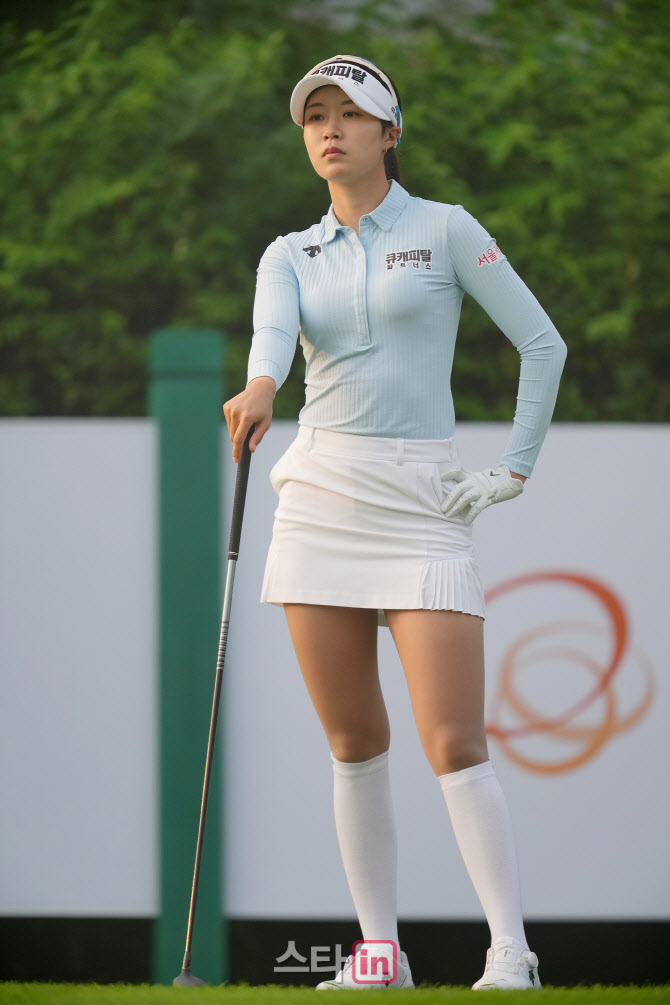This professional photograph captures a young, athletic South Korean golfer intently studying her next shot on a golf course. Dressed in a coordinated golfing outfit, she dons a white visor, a long-sleeved green or blue button-up shirt, and a stylish white mini skirt. Her attire is completed with white knee-high socks and white golf shoes. The golfer stands with her left hand on her hip while leaning slightly on her putter with her right hand, showcasing her focused demeanor. A golf glove on her left hand hints at her readiness for action. The background features trees, a fence with an interesting symbol, and a broadcast logo in Japanese, contributing to the professional and possibly sponsored event setting.